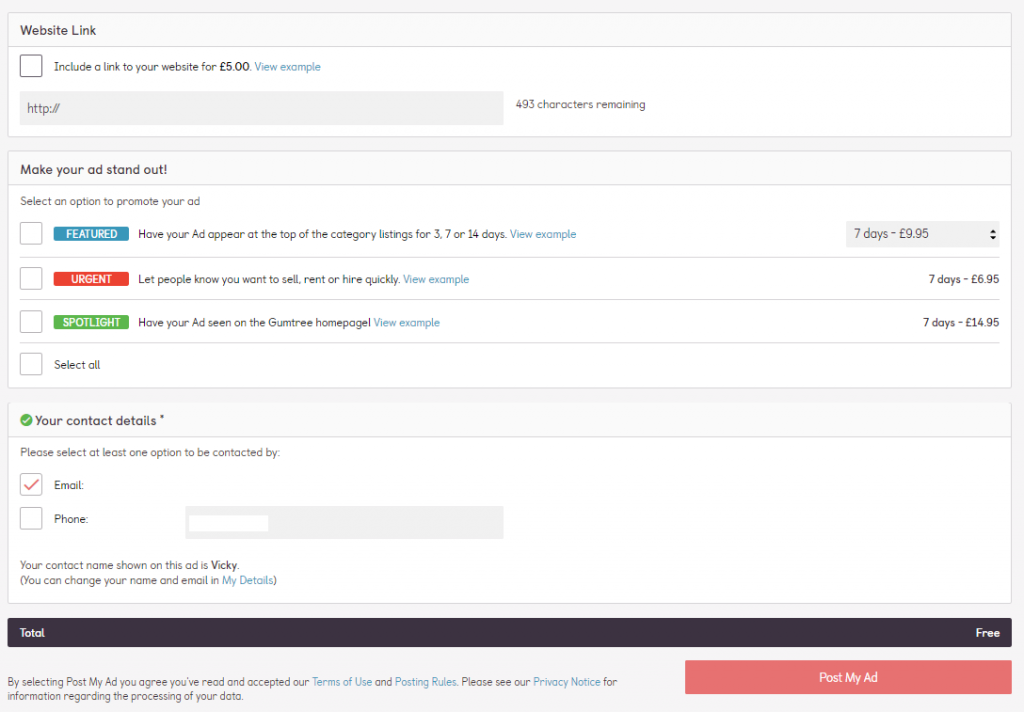The image depicts a detailed form for posting an advertisement, featuring various options and instructions against a light purple background.

At the top, there is a light purple header that reads "Website Link." Below this header, a light-colored box includes a smaller box with text that says, "Include a link to your website for €5." An example button is also present. Adjacent to this, a small purple box displays "HTTP," and beside it, two lines indicate the available characters, showing "493 characters remaining."

Further down, another purple section prompts, "Make Your Ad Stand Out!" Inside this section, there is a large white box subdivided into four smaller options:
- The first option, indicated with a blue label "Featured," suggests featuring your ad at the top of category listings for 3, 7, or 14 days. A sample link and pricing for "7 days for $9.95" is accompanied by up and down selection arrows.
- The second option, marked with a red "Urgent" label, advises letting potential buyers know you want to sell, rent, or hire quickly. An example link and "7 days for $6.95" are provided.
- The third option, labeled "Spotlight" in green, promotes displaying your ad on the Gumtree homepage. An example link and "7 days for $14.95" accompany this option.
- Lastly, there is a "Select All" box for convenience.

Continuing down, another blue section with a green circle and a check mark reads "Your Contact Details" with an asterisk denoting required information. In a larger white box, the instructions ask to select at least one option for contact preference. Options include "Email" and "Phone," with the Email option already checked by a red tick. Additional details include the contact name, listed as "Vicki," with a note that it can be changed in the "My Details" section.

At the bottom, a black box displays the "Total" cost as "Free." A statement below clarifies that by posting the ad, you agree to the terms of use and posting rules, and provides a link to the privacy notice. Finally, a pink button at the very bottom reads "Post My Ad."